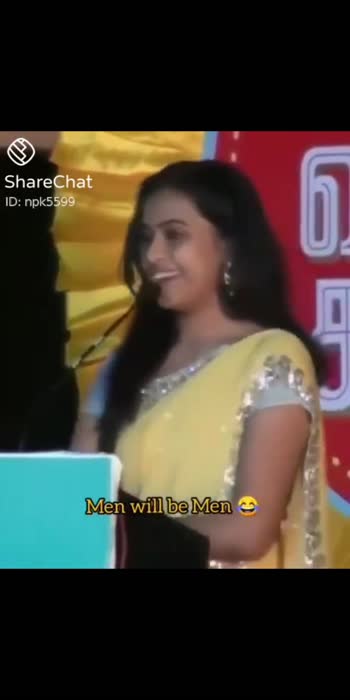The image is a screenshot resembling a Snapchat capture featuring an Indian woman with dark skin and long black hair that flows down to her breasts. She is facing slightly to the left, smiling and laughing. The woman is dressed in a beautiful yellow sari adorned with silver trim and appears to be wearing earrings that can slightly be seen beneath her hair. In front of her, text in yellow states, “Men will be men,” with the first letters of "Men" capitalized and accompanied by a laughing, crying emoji. The photograph is bordered by thick black horizontal bars at the top and bottom. 

At the top left corner below the black band, a symbol and the words "Share Chat" are written in white, accompanied by a white ID number. Behind the woman, there appears to be a banner with gold fringe, featuring a section of red with white symbols and another section in yellow. On the bottom left of the image, there's a light blue square. Additionally, a black foam microphone on a black stick is positioned near her.